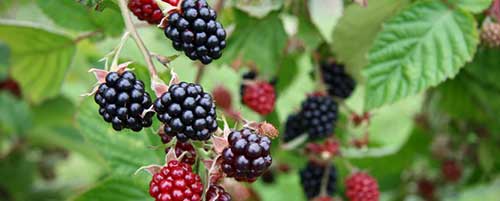This closeup photo captures a vibrant array of berries on a bush with serrated leaves. Predominantly, there are plump, realistic-looking berries on a beige-green vine. The berries exhibit a spectrum of colors—ranging from deep, almost black purples and blue-black hues to bright maroon and vivid apple red tones. The vividness of the berries contrasts with the background, which is slightly out of focus and contains various green leaves, some darker and others lighter, with one leaf showing signs of insect activity. The foreground prominently features three very ripe, almost blackish-blue berries and another purple berry that is not yet fully ripe, alongside two strikingly shiny red berries. The light accentuates these foreground berries, making them appear almost tangible, as if you could reach out and pick them. The background is adorned with additional blue and red berries, though they are more muted and blurred, adding depth to the image.